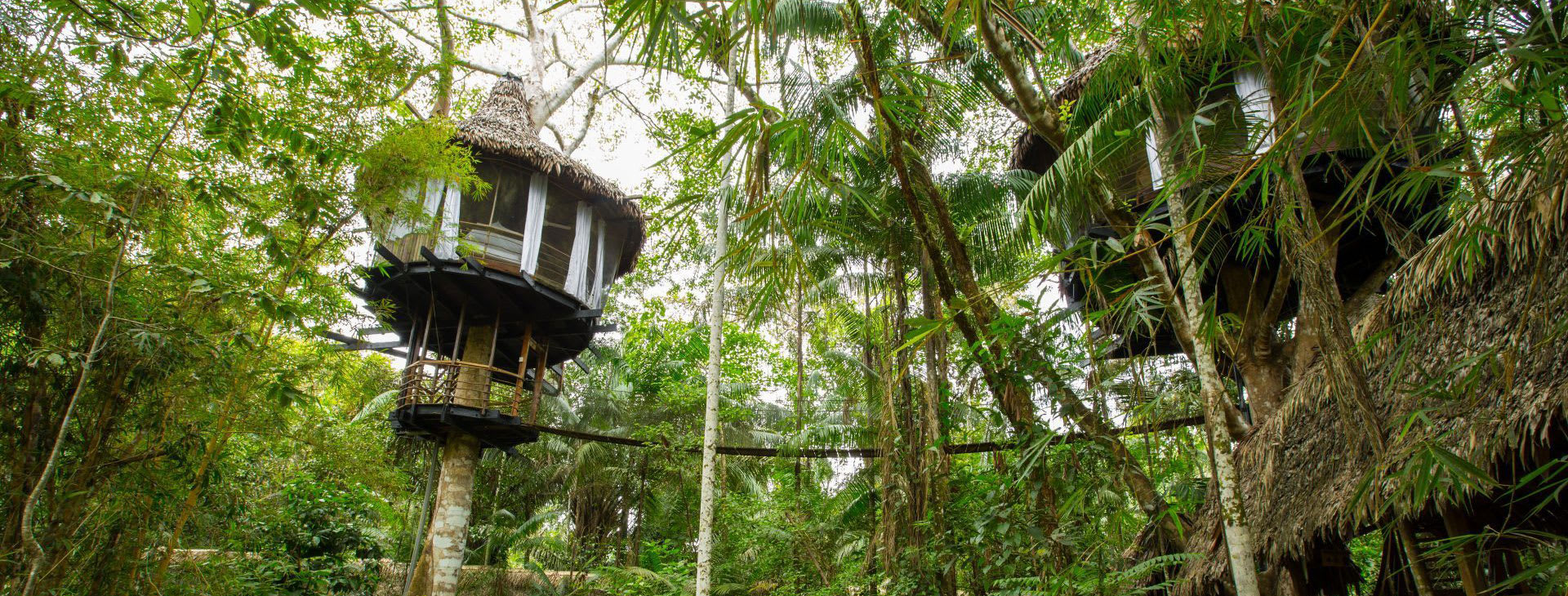The photograph captures a pair of treehouses nestled within a dense, verdant forest composed of tall, narrow trees with both full and skinny leaves. The scene is set from a ground perspective, gazing up at the canopy where the treehouses are perched. The primary treehouse on the left features a base with climbing ropes and a balcony-like rope arrangement. Its circular design includes windows and a roof constructed from straw, resembling a grass-topped hut. The treehouse to the right is partially obscured by the plentiful leaves but remains discernible. There is a bridge connecting the two treehouses, adding cohesion to the aerial dwellings. White curtains drape from the structures, enhancing their homey appearance, suggesting they might serve as unique accommodations or even an Airbnb. Blue sky peeks through the dense foliage, illuminating the lush greenery and adding depth to this secluded arboreal habitat.